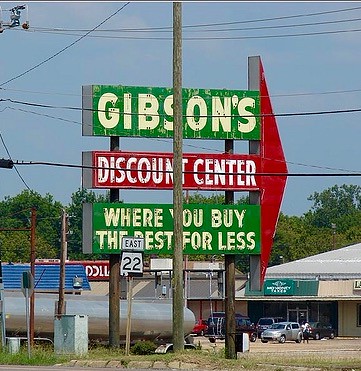The image captures an outdoor scene under a blue sky with wisps of white clouds. Dominating the center is a tall, brown pole. Affixed to the pole is a sign prominently displaying the text "Gibson's Discount Center" with a red arrow pointing to the right. Below, in smaller text, it states, "where you buy the best for less." A street sign in front of the main sign reads "East" in black letters, positioned above a black number "22." In the background, a cluster of buildings completes the scene.